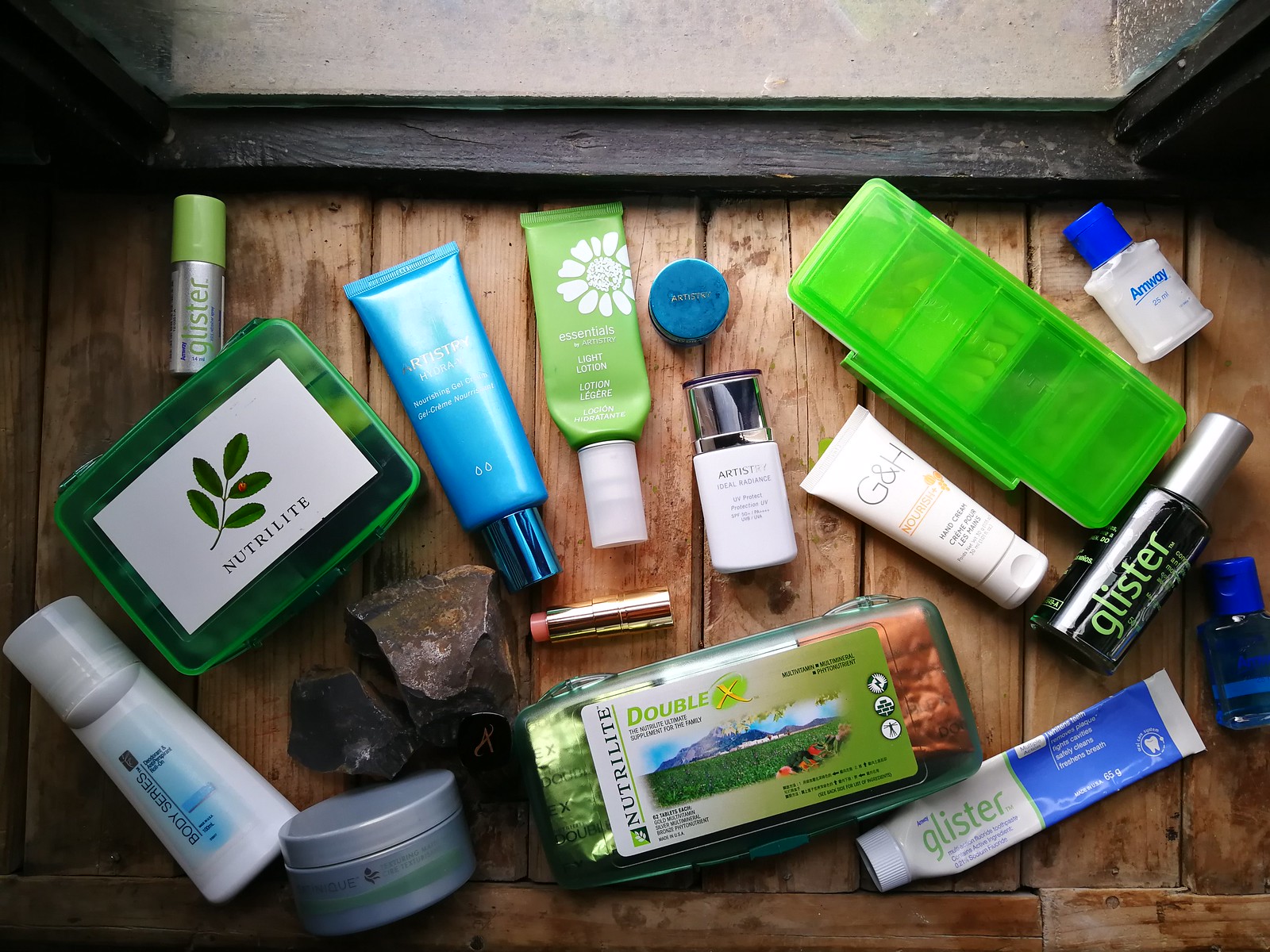The photograph offers a bird's-eye view of a weathered wooden deck, its boards showing significant signs of wear and tear, likely from prolonged exposure to water. The deck's surface, once finished, now displays numerous water stains and patches where the finish has eroded. At the top edge of the image, a black wooden frame, likely a window, partially reveals a concrete surface beyond.

Scattered across the deck are various toiletry items. On the right side of the frame, a black tube with a silver cap bears the green inscription "GLISTER." Below it lies a white tube also marked "GLISTER" in green, featuring a blue band across the majority of the tube and a white cap. Adjacent to these, a small green plastic container is labeled "NEUTRALIGHT DOUBLE." Additionally, the scene includes a gray jar with a screw top, among other miscellaneous containers, including one resembling a lipstick tube. The assortment of products adds a cluttered yet intriguing element to the rustic setting.